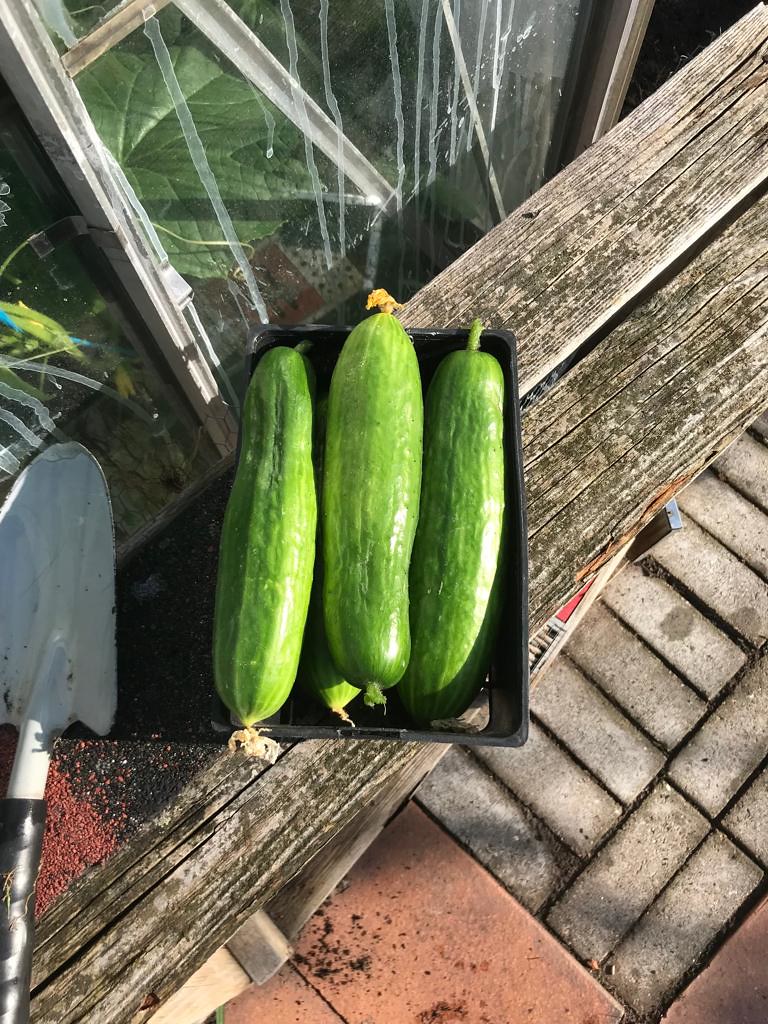This is a detailed color photograph capturing a quaint garden scene focused on freshly harvested vegetables. Centered on a weathered, stained wooden workbench is a small black tray holding four or five plump and shiny cucumbers, each displaying a green hue with glints of light reflecting off their surfaces, as well as some remnants of dead flowers. To the left of the tray lies a white-bladed garden trowel with a dark handle, resting on a sprinkling of a red substance. The background reveals a greenhouse window streaked with numerous white drippings, through which lush green leaves from growing plants are visible. Below the workbench, the ground features a mix of gray and red block paving with scattered dirt, adding to the rustic charm of the garden workspace.